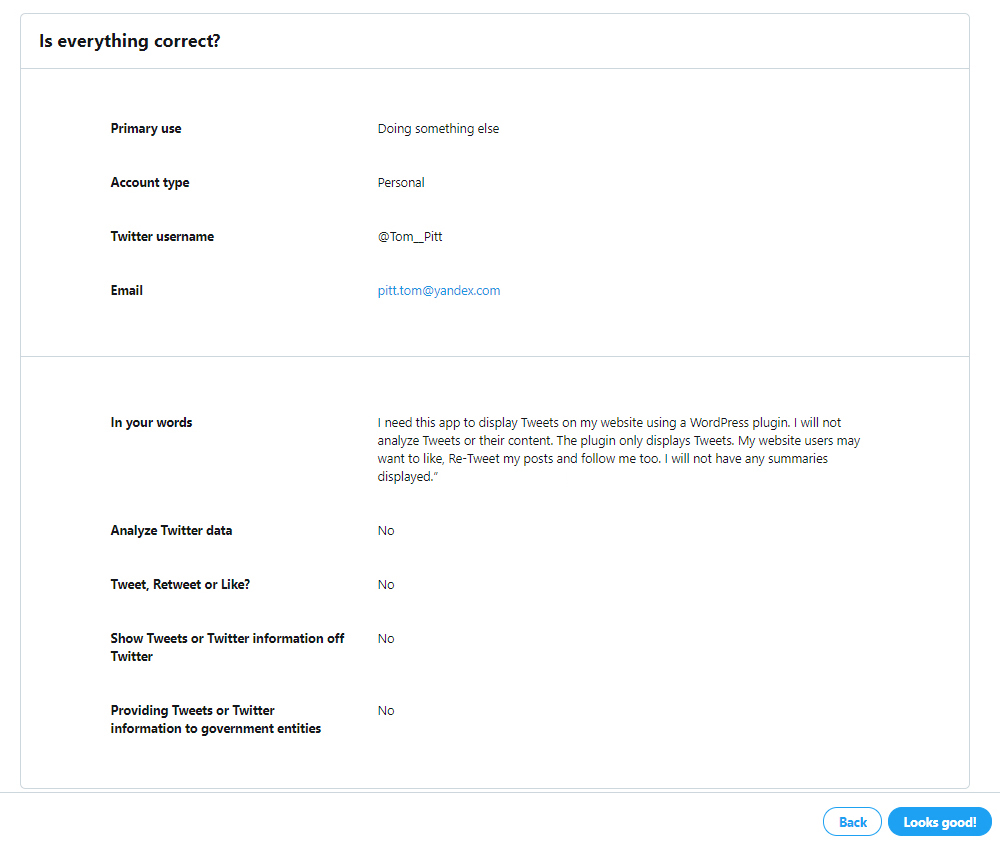This image showcases a screenshot of a form or application interface, predominantly positioned in the upper left corner. The header of the form reads "Is everything correct?" Below this header, various sections are filled out with user information and intended usage declarations.

The first section details the primary use and account information:
- **Primary Use**: Doing something else
- **Account Type**: Personal
- **Twitter Username**: @tom__pit
- **Email**: pit.tom@yandex.com

Following this, there is a section titled "In Your Words" where the user elaborates on their intended use of the app:
- **User Statement**: "I need this app to display tweets on my website using a WordPress plugin. I will not analyze tweets or their content. The plugin only displays tweets. My website users may want to like, retweet my posts, and follow me too. I will not have any summaries displayed."

Next, a series of statements with simple yes or no answers outline the user's commitments regarding the usage of Twitter data:
- **Analyze Twitter Data**: No
- **Tweet, Retweet, or Like**: No
- **Show Tweets or Twitter Information off Twitter**: No
- **Providing Tweets or Twitter Information to Government Entities**: No

In the bottom right corner of the screenshot, there are two buttons:
- The left button is labeled "Back."
- The right button is labeled "Looks good."

This detailed screenshot appears to be a crucial step in verifying user intent and compliance within the application's setup or approval process.